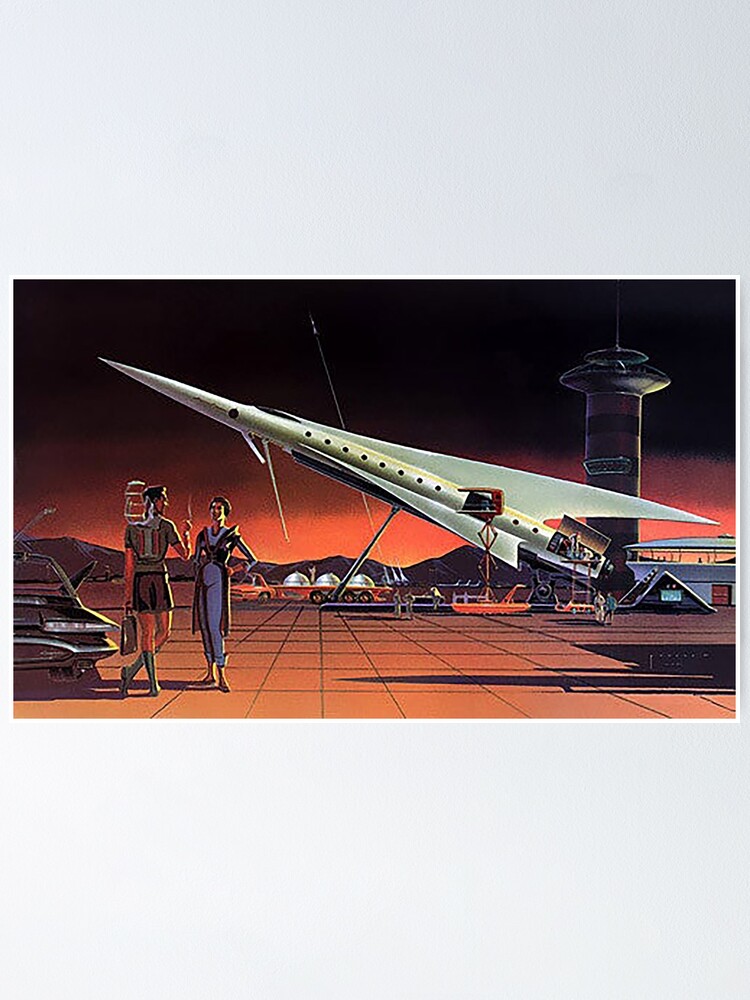This detailed illustration, evocative of a 1950s comic book style yet rendered with a more realistic touch, depicts a futuristic airport scene at sunset. Dominated by an orange sky that fades into black, the picture features a sleek, modern-looking white rocket ship aircraft with red details, poised at an angle as if ready for takeoff. To the right of the aircraft stands a black air traffic control tower.

In the foreground on the left, a man in brown shorts and a khaki-colored shirt, with green socks peeking out, converses with a woman dressed in a blue pantsuit. They are next to a futuristic drivable vehicle, possibly a cart designed for airport use. The tarmac they stand on is tiled with orange squares.

Further back, a tanker truck or perhaps an orange vehicle towing three dome-like objects is visible. There are also small, indistinct figures moving near the plane, adding to the bustling feel of the airport scene. Overall, the illustration captures a blend of mid-century imagination and futuristic elements, bringing to life a moment just as day turns to night.